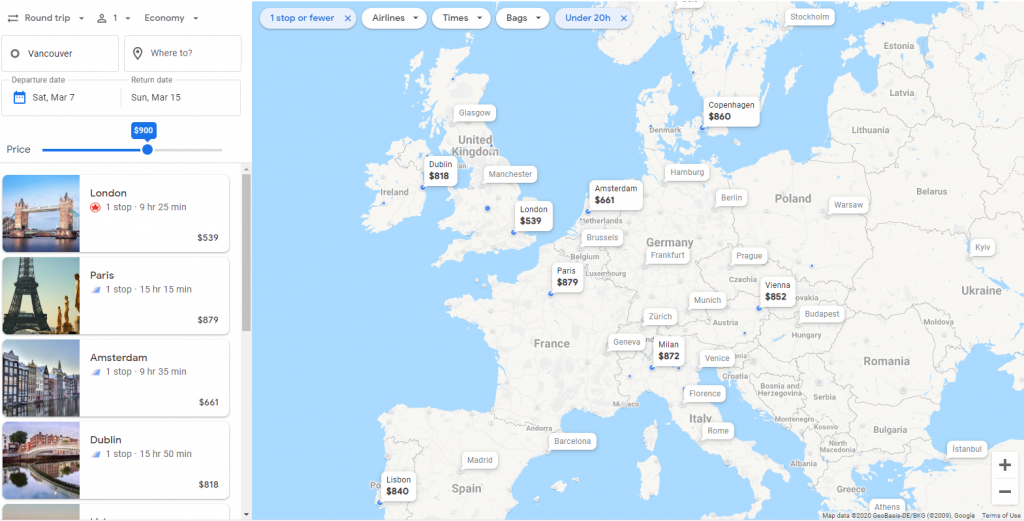The image depicts a computer screen displaying a flight booking website. On the left side of the screen, options for flights to London, Paris, Amsterdam, and Dublin are listed. The search criteria above indicate a round trip for one person in the economy class. The departure city is Vancouver, but the destination has not been entered yet. The departure date is set for Saturday, March 7th, with a return on Sunday, March 15th. Below these details, a price range is visible, currently showing $900, with a scroll bar for adjusting to view potentially lower or higher prices. In the background, a map of Europe is visible, shaded in gray, with several blue dots indicating different cities. Each dot has a small speech bubble showing the flight prices to those destinations.